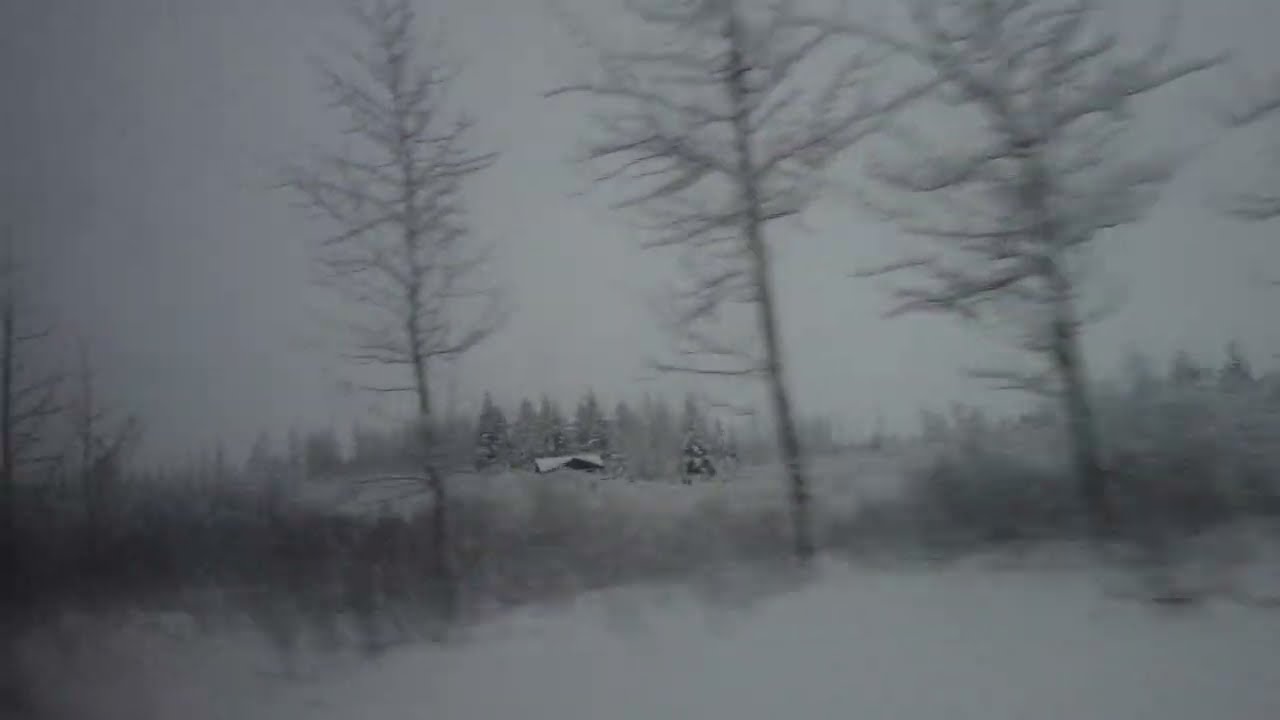In this low-resolution, photorealistic winter forest scene, the ground is blanketed in snow, rendering it a solid, uninterrupted white. The foreground contains several barren deciduous trees and plants, dark brown and stick-like in appearance, lacking any foliage. Between these trees, sparse brush sticks up to about a foot high, its color blending into the wintery palette. A small house, partially obscured and situated just left of the image center, features a snow-covered arched roof. Surrounding the house are tall, cone-shaped evergreen trees, their branches weighed down with snow yet hinting at the green beneath. The sky stretches overhead, a heavy gray that grows darker toward the upper left corner, casting a muted tone over the entire scene, devoid of vibrant colors.